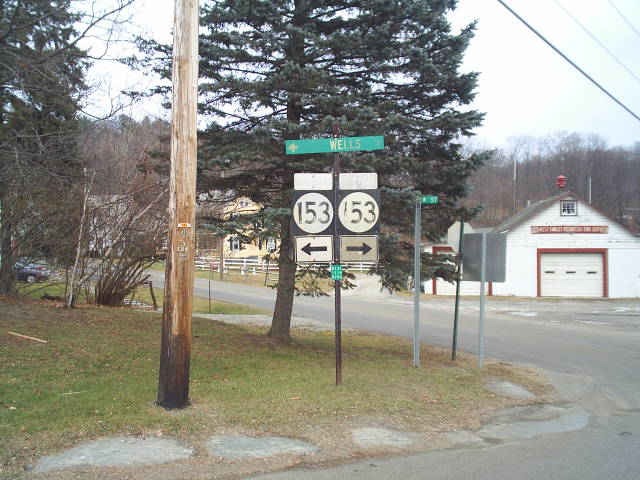The image depicts a rural residential street corner, characterized by a small patch of green grass bordered by a worn, light gray stone boulevard. Prominently to the left stands a weathered power pole, blackened at the base and fading to light at the top. Adjacent to this pole, a collection of street signs on metallic stakes draw attention. At the top, a green rectangular sign displays the word "WELLS" with an arrow pointing left. Below it, two black and white signs feature a central white circle with the number "153" in black, each accompanied by arrows pointing in opposite directions—left on the left side, right on the right side. The street itself is paved in light gray.

Beyond the signage, a tall pine tree stretches into the sky. To the right of the tree stands a red and white building, identifiable by its large garage door and striking red chimney. The context suggests a quiet, less trafficked area, possibly where homes or small businesses are situated. The vantage point of the photograph is at ground level, likely taken by someone standing on the road rather than inside a vehicle. The overall scene is serene, reflecting the understated charm of a rural neighborhood intersection.